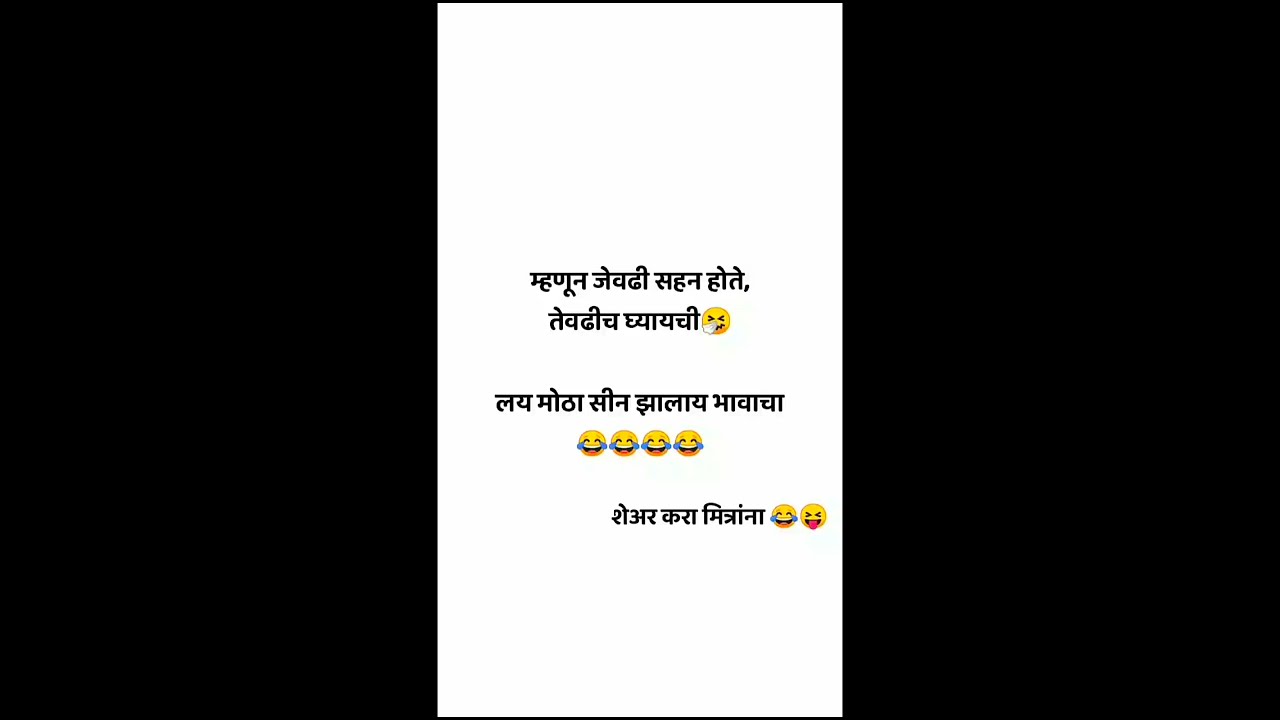The image depicts a rectangular panel that is wider than it is tall, with a 2:1 width-to-height ratio. The panel is divided into three sections: the left and right sections are black rectangles, framing the central white panel. In the central panel, there is black text written in an unknown script resembling Middle Eastern or Indian characters, formed by a series of lines and curves connected by a horizontal bar at the top of most words. The text is arranged into five lines, with the specific formatting of each line including various emojis:

1. The first line ends with a sneezing emoji.
2. The second line ends with a sneezing emoji, as reiterated, though more clearly it shows a pattern of ending in such an emoji.
3. The third line contains no emojis.
4. The fourth line is filled with four crying laughing emojis.
5. The final line concludes with both a crying laughing emoji and a squinting tongue-out emoji.

The detailed placement and type of emojis closely accompany the lines of the black script on the central white panel, framed by the thick black bars on either side.